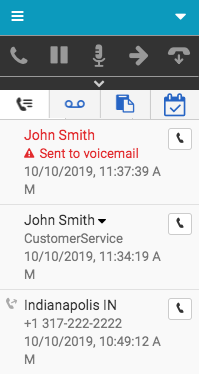The image appears to be a screenshot of a smartphone interface, possibly displaying a call log or contact details. At the very top, there is a blue bar with three horizontal white lines on the left-hand side and a white downward arrow on the right-hand side. Below this, there is a black section with a series of gray icons: a phone icon, two vertical lines, a microphone icon, an arrow pointing to the right, and an arrow pointing down with a telephone symbol. 

Centered below this, there is a gray arrow. The screen then transitions to a white background with four top-aligned icons in boxed sections: a telephone icon, two circles with a line under them, a clipboard with paper overlapping it, and a file with a blue check mark. Below these icons, in red text, is the name "John Smith," accompanied by a triangle with an exclamation point and the notation "sent to voicemail" next to a gray-outlined phone icon. 

Under the "sent to voicemail" message, there is the date and time "10/10/2019, 11:37:39 AM" written in gray. Below that, "John Smith" is repeated in gray text with an arrow pointing downward. Faintly below this, it says "customer service" followed by the same date but a different time, "10/10/2019, 11:34:19 AM," again with an "AM" suffix indicating the time. Another gray-outlined telephone icon is next to John Smith's name.

Further down, there is a black text showing "Indianapolis, Indiana" with a telephone icon and an arrow on the left. Under the city name, a phone number is listed as "+1 317-222-2222". Below the phone number, another date and time are displayed: "10/10/2019, 10:49:12 AM" along with an "M" and a gray-outlined telephone icon adjacent to "Indianapolis, Indiana".